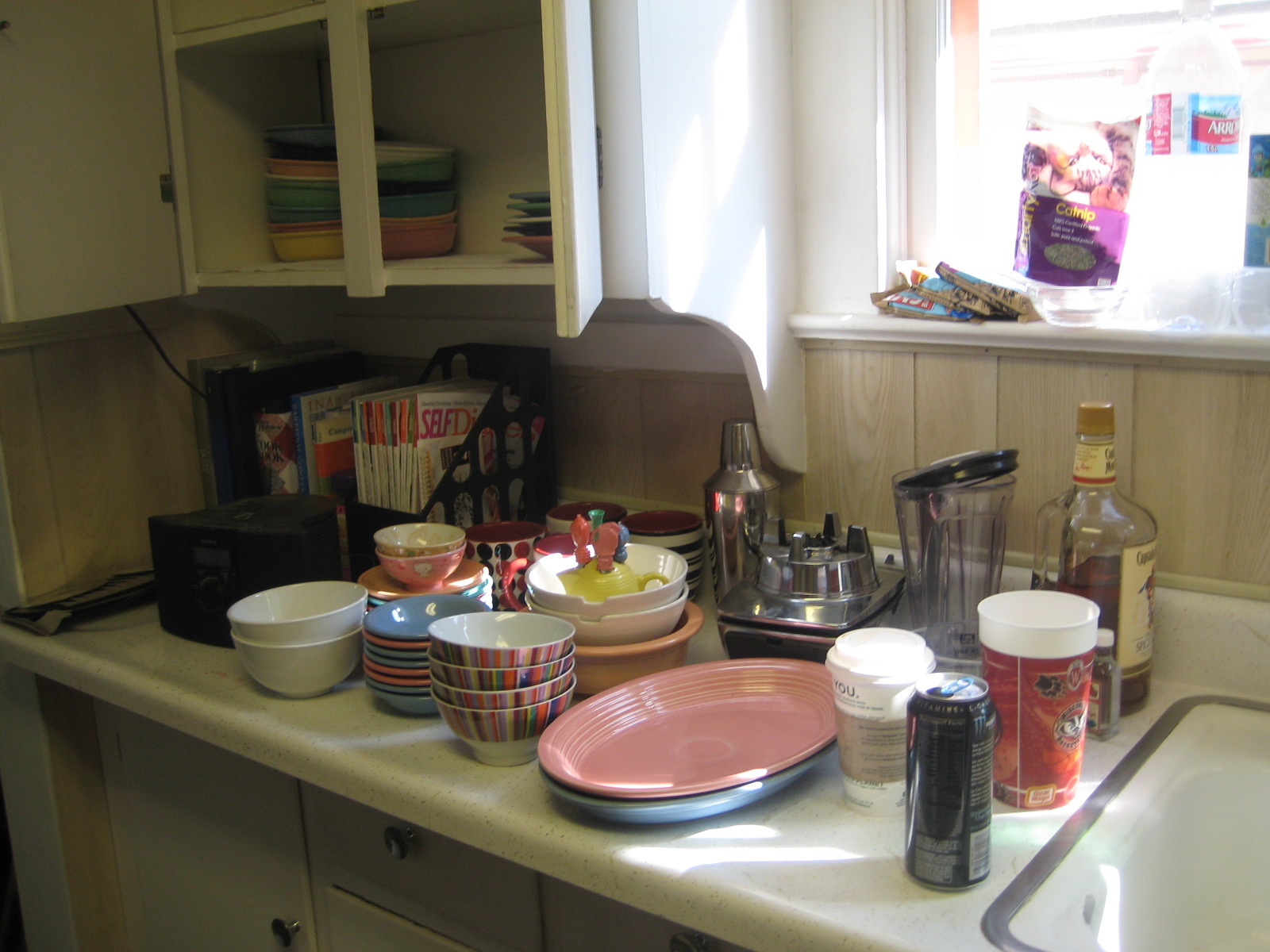A cozy home kitchen bathed in daylight features white cabinets with open doors revealing stacks of colorful mini bowls and the edges of various plates. To the right of the cabinets, a window lets in abundant sunshine, illuminating the vertical light wood paneling on the walls. The off-white, speckled countertop hosts an array of items, including a large bottle of water and a package of catnip on the window ledge. Below the countertop, white cabinets and drawers add to the clean, bright aesthetic. 

On the counter, just to the right, sits a stainless steel banded sink with a white basin. The counter is cluttered with a captivating mix of objects: a large bottle of Captain Morgan, a blender, two large oval plates, several more bowls, and an assortment of cups. Magazine racks filled with magazines, a coffee cup with a lid, a tall plastic cup, and a can of Monster Energy drink complete the scene, reflecting the kitchen’s blend of functionality and homey charm.